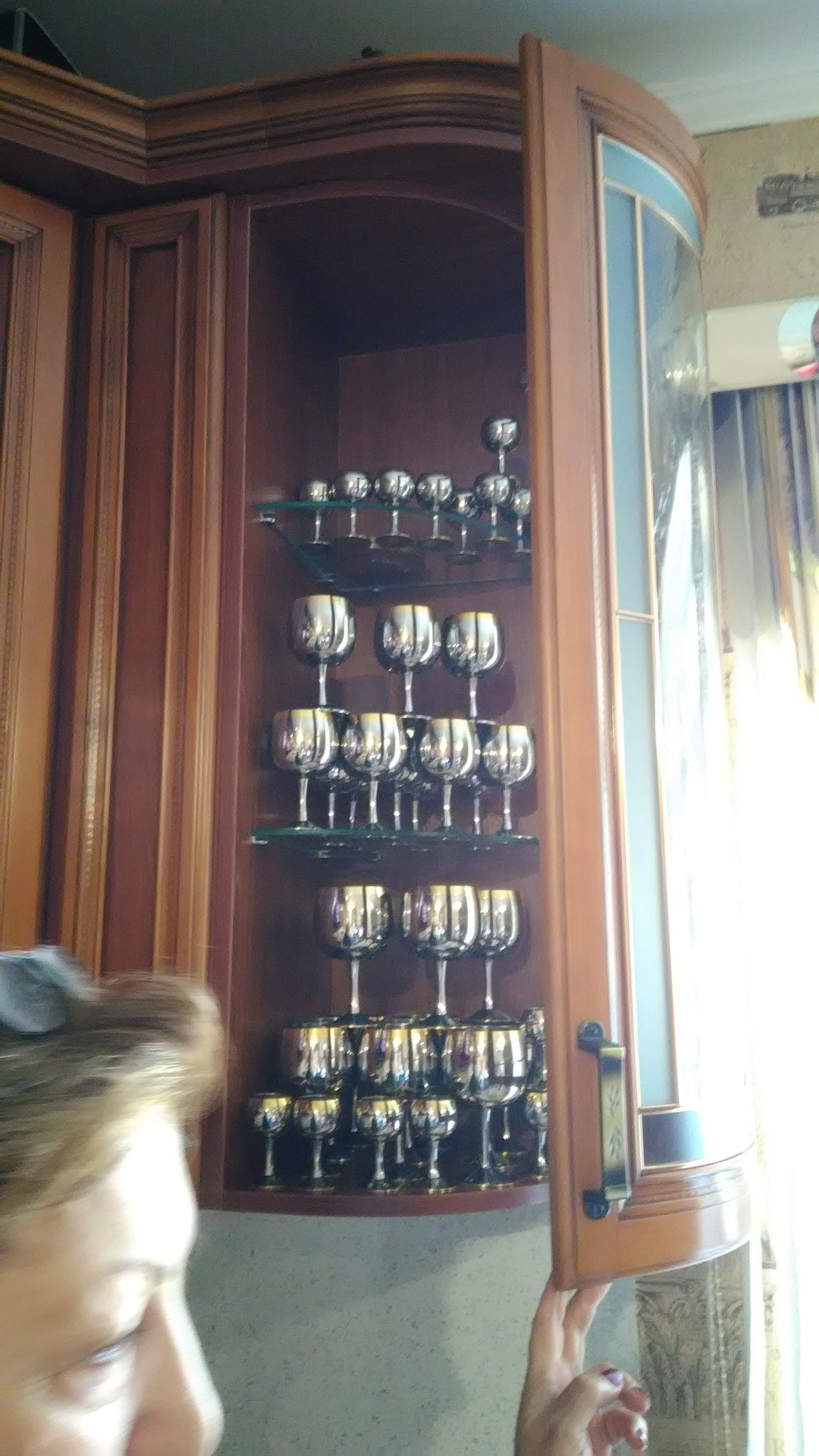This image depicts a glass-fronted, round end cabinet with a wood frame, positioned in a corner of a kitchen. The cabinet door, which has a brass handle, is slightly open, revealing its content. Inside, there are three glass shelves, each shaped like a triangle with the point fitting into the cabinet's corner. 

The bottom shelf holds a collection of neatly stacked silver chalices or small wine glasses. The middle shelf contains a smaller set of silver goblets, while the top shelf showcases an even smaller set of similar silver glasses. All the goblets share the same style but vary in size, from larger ones on the bottom shelf to the smallest on the top.

A woman with brown hair, wearing glasses on top of her head, is seen pushing open the glass door. She has a fair complexion, and from the sunlight streaming into the house, it appears to be a bright day. The woman's face is partially visible towards the bottom left corner of the image, adding a personal touch to the scene.